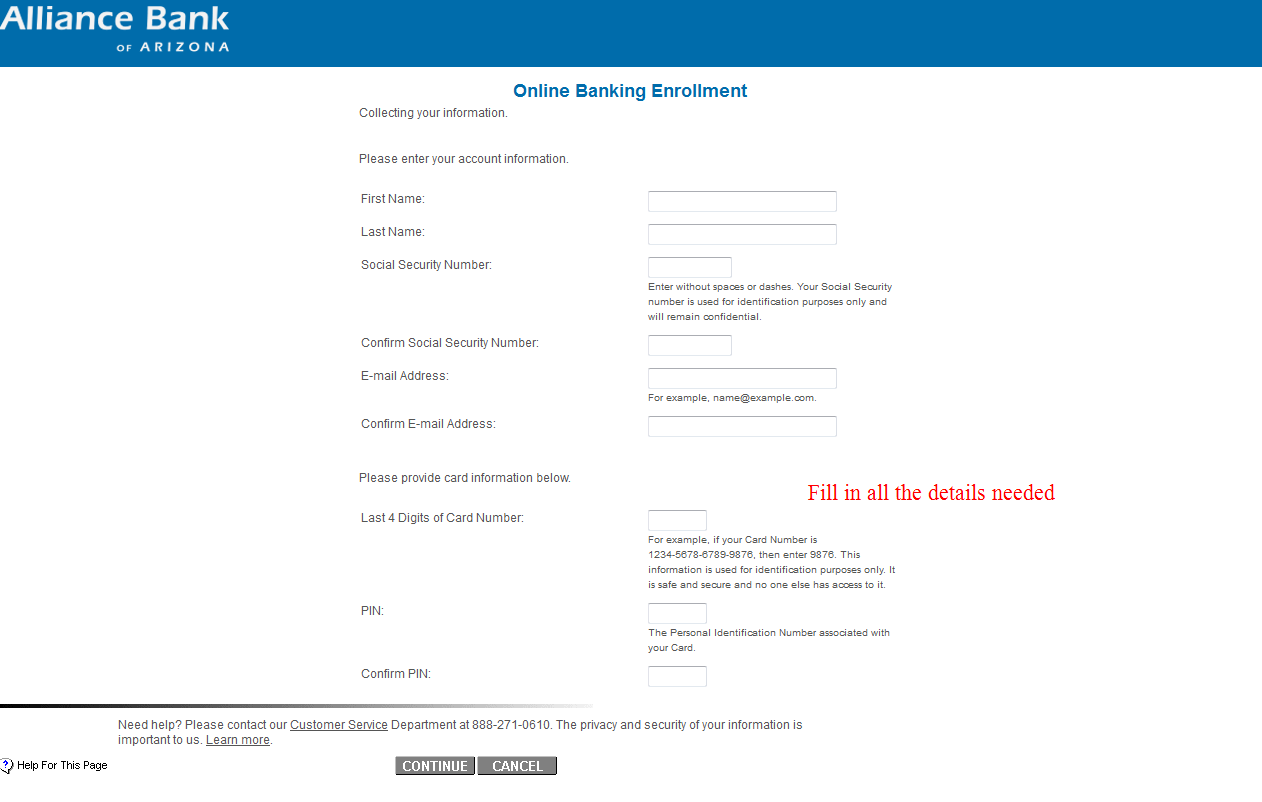The image is a screenshot of a website focused on online banking enrollment for Alliance Bank of Arizona. 

At the top, there is a medium to dark blue banner containing the bank's name in white text on the left: "Alliance Bank of Arizona," with 'Alliance' and 'Bank' capitalized. Below this banner, on a white background, the title "Online Banking Enrollment" is prominently centered in blue text, with each word starting with a capital letter.

The page proceeds with instructional text in black that states "Collecting Your Information" and a prompt: "Please Enter Your Account Information." Below this, there are designated fields for user input:

1. First Name: followed by an input field.
2. Last Name: followed by an input field.
3. Social Security Number: includes a note in italics reminding users to "Enter Without Space or Dashes." A disclaimer follows, stating, "Your Social Security Number is used for identification purposes only and will remain confidential."
4. Confirm Social Security Number: followed by a corresponding input field.
5. Email Address: followed by an input field.
6. Confirm Email Address: followed by an input field.

The page then instructs users to "Please Provide Card Information Below" and lists:

1. Last four digits of card number: accompanied by an input field and highlighted in a pinkish red tint.
2. A notice in the same pinkish red color that says "Fill in All the Details Needed."
3. Fields for PIN Number and Confirm PIN: each followed by an input field.

At the bottom of the page, there is a section for those needing assistance. It reads: "Need Help? Please Contact Our Customer Service" followed by a telephone number for support. Lastly, there are two buttons: "Continue" and "Cancel," allowing users to proceed or exit the enrollment process, respectively.